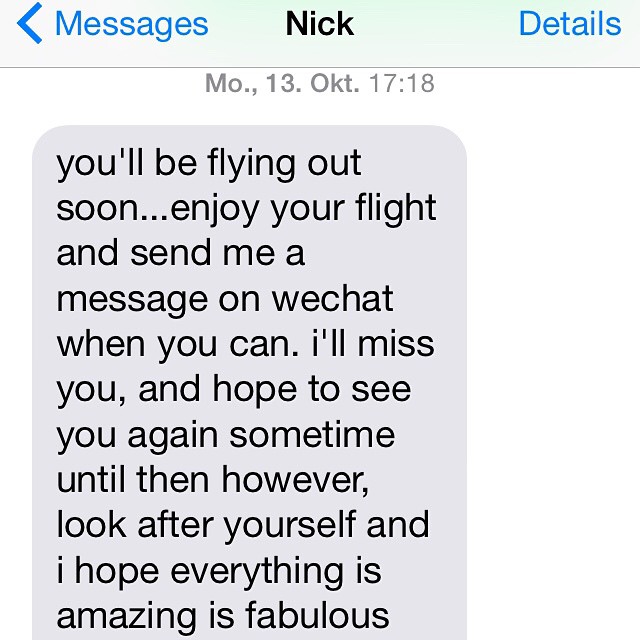This is a screen capture of a chat message on a smartphone. At the top of the screen is a light green bar with "Messages" in black on the left, "Nick" in bold in the center, and "Details" in blue on the right. Below this bar, the date and time are displayed as "MO, 13 OKT, 1718". The main message is in black text on a gray background, reading: "You'll be flying out soon. Enjoy your flight and send me a message on WeChat when you can. I'll miss you and hope to see you again sometime. Until then, however, look after yourself and I hope everything is amazing and fabulous."